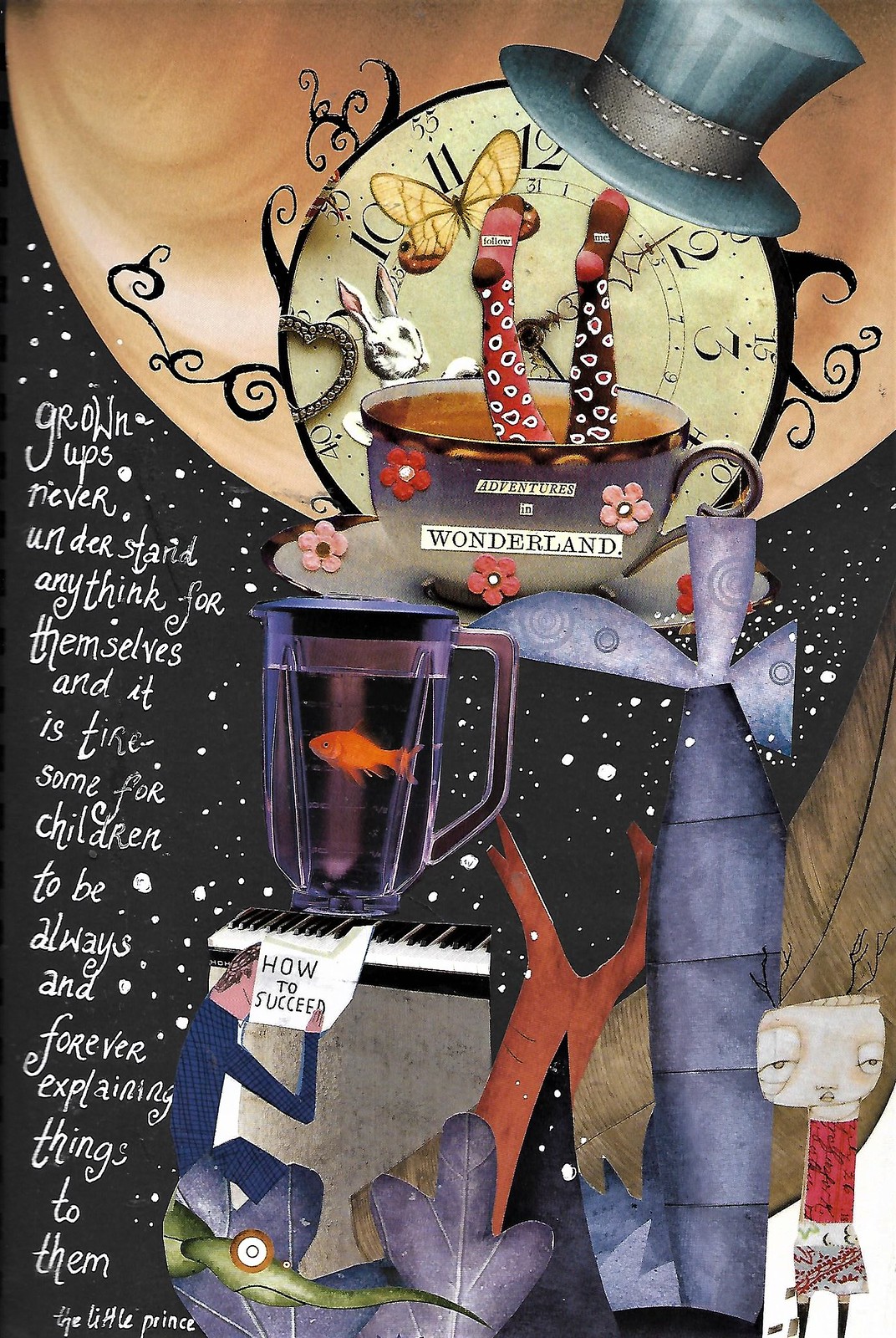This intricate surrealist art collage, presented in portrait orientation against a black, star-speckled background, integrates vivid imagery from classic literature and imaginative elements. At the upper part of the image, an antique pocket watch featuring dark, tentacle-like scrolls is adorned with an aqua top hat and hosts a yellow-orange butterfly and a white rabbit with misshapen ears. The watch overlays a pale, beige planet and below it, a teacup with the phrase "ADVENTURES IN WONDERLAND" emerges, with the tea or coffee within sprouting legs in colorful, spotted hose.

On the lower part, a piano keyboard anchors the scene, before which a man in blue clothes holds a sign reading "HOW TO SUCCEED." Accompanying this are aquatic-themed decorations, such as floating plants, a goldfish inside a blender container, and a blue, possibly submarine-like object. To the right, a somber child appears in an orange shirt and multicolored shorts. The left side of the image is framed by white text stating, "Grown-ups never understand anything for themselves, and it is tiresome for children to be always and forever explaining things to them," credited to "The Little Prince." This collage blends elements of whimsy and reflection, creating a rich tapestry reminiscent of "Alice in Wonderland" and further deepened by literary allusions.